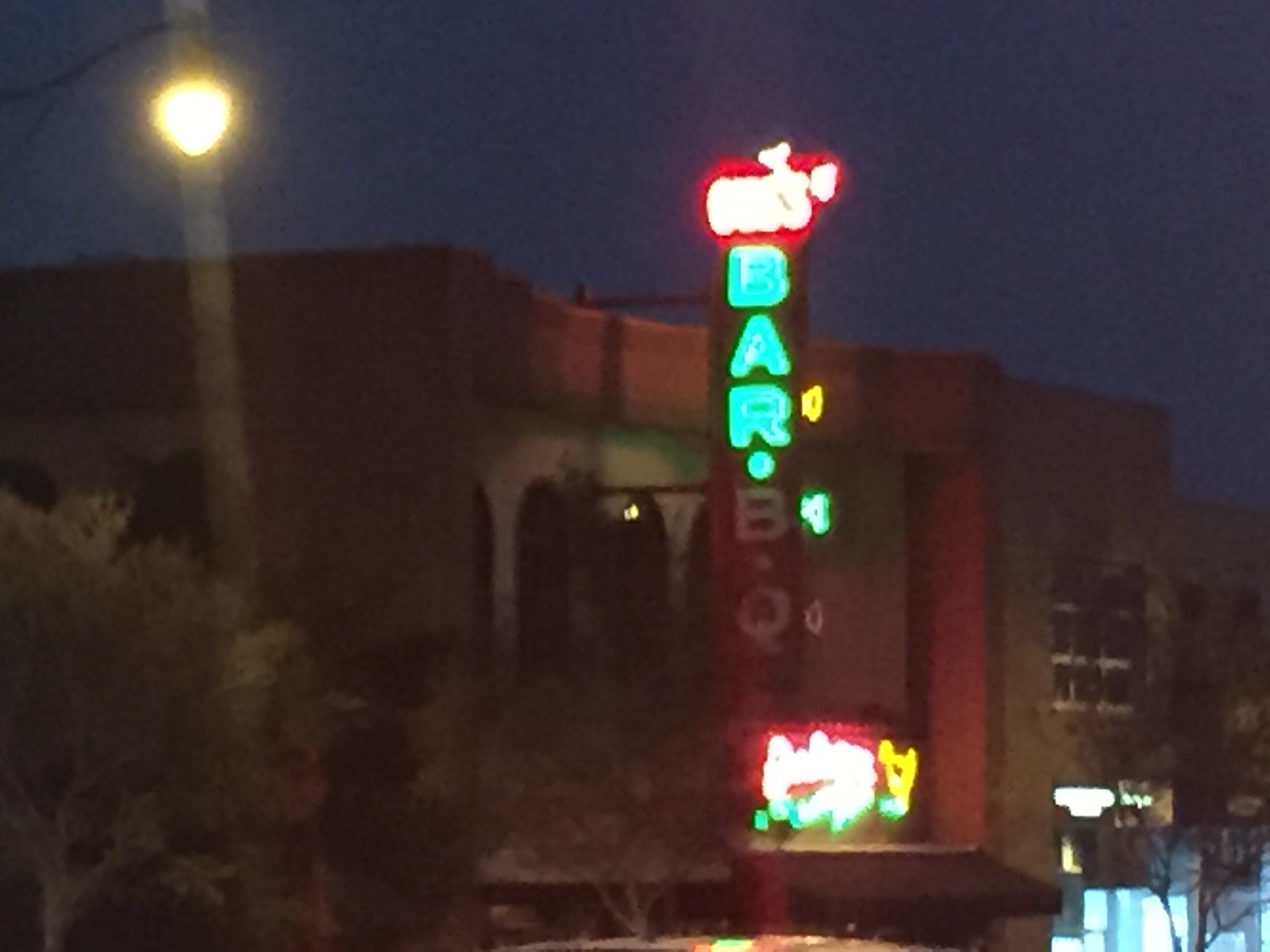This photograph, taken outdoors at nighttime, depicts a dimly lit red brick or stone building believed to be a bar or restaurant. The building features a couple of windows, and a vertical neon sign mounted on metal rails that says "BAR" in blue neon letters, though some descriptions suggest it could be neon green. Below this sign is another partially visible neon sign, the text of which is illegible. To the left side of the photo, a tree with leaves is present, while another tree is partially visible to the right. The sky is a dark blue, and in the upper left corner, a bright street lamp casts a globe of light, illuminating the scene.